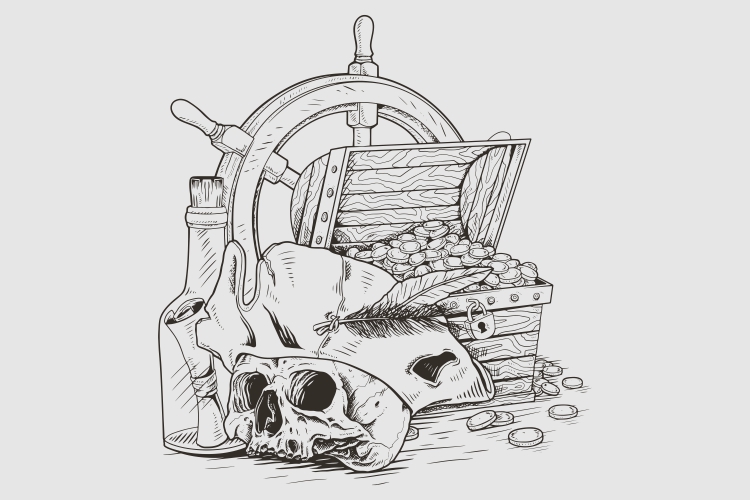This black and white illustration depicts several iconic pirate-related objects against a light gray background, arranged centrally within a rectangular frame that is wider than it is tall. At the back, a ship's wheel with two visible rounded spokes anchors the composition. Slightly to the right and in front of the wheel is an open treasure chest with a curved top, made from swirled wooden planks. The chest overflows with round coins, some of which have spilled onto the ground. A rounded lock with a prominent black keyhole dangles from the front of the chest. Positioned to the left of the treasure chest, a skull missing its lower jaw glares out with deep black eye sockets and a nose hole. This skull is adorned with a worn, triangular pirate captain's hat featuring a single feather in front. Just behind the hat and slightly to the left, a glass bottle sealed with a light-colored cork contains a rolled-up, tied piece of paper. The intricate details of the objects, from the swirls in the wooden chest to the feather in the pirate hat, bring the sketch to life, creating a vivid tableau of pirate lore.